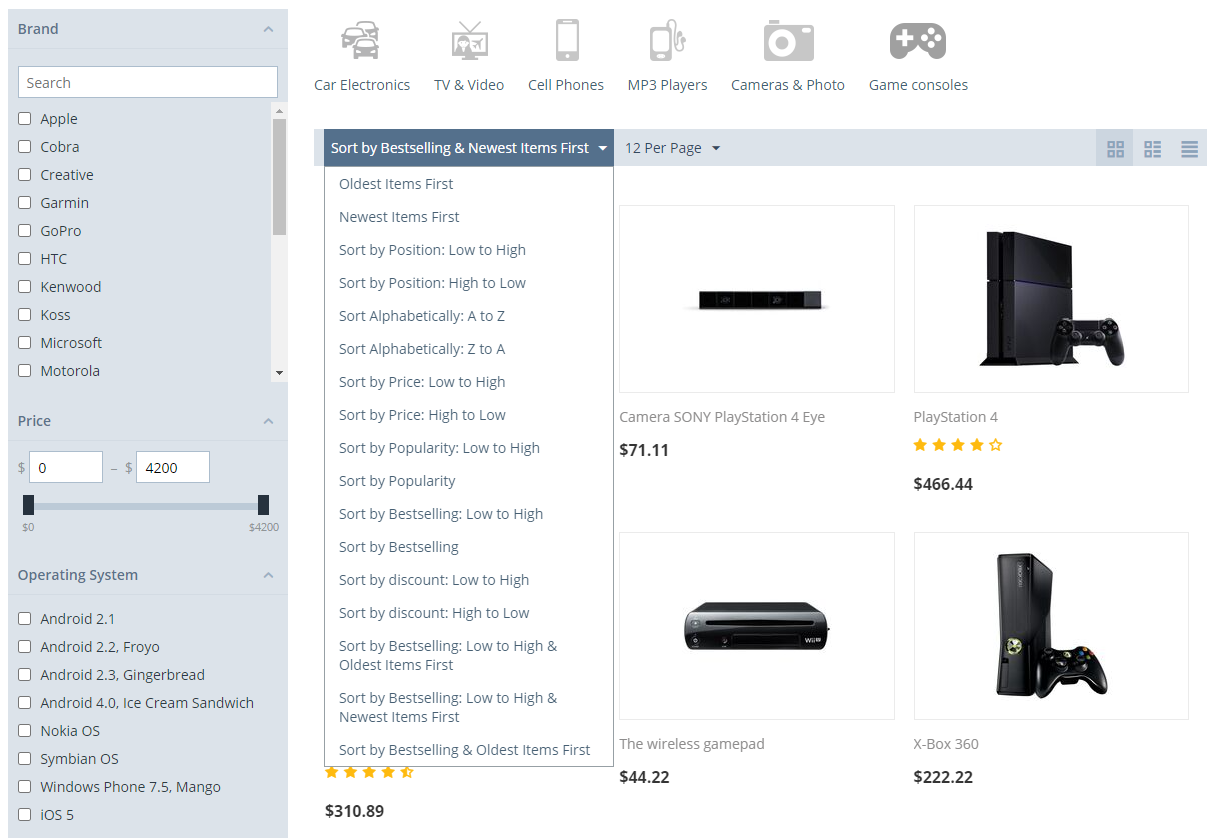The image displays a detailed inventory list organized into a column. The list includes 10 boxes, each labeled with different brands and items: Apple, Cobra, Creative, Garmin, GoPro, HTC, Camera, Cosmos, Microsoft, and Motorola. Additionally, the price range for these items is shown as 0 to 4200. The supported operating systems mentioned are Android 2.1, Android 2.2, Android 4.0, Android 2.3 (Gingerbread), Android 4.0 (Ice Cream Sandwich), Nokia OS, Symbian OS, Windows Phone 7, Amiga, and iOS 5. Categories listed alongside these include car electronics, TV and videos, cell phones, 3-pose cameras, photo, game consoles, Neewer products, and Sony Xperia.